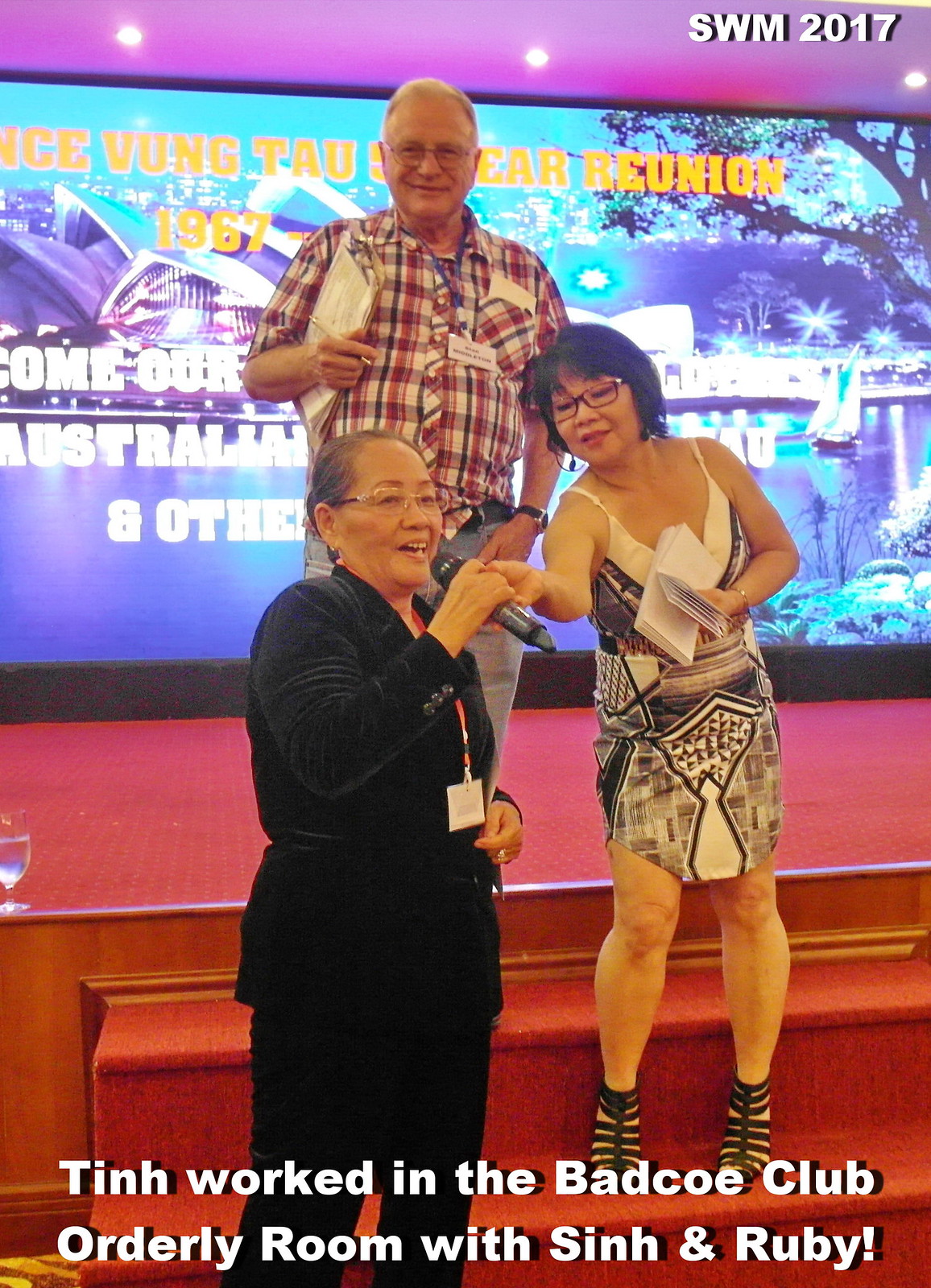In the image, three people are standing on a stage characterized by two red steps. At the forefront, there's a woman wearing a black suit, glasses, and a lanyard, speaking into a microphone. She stands on the ground level of the stage. Appearing to assist her, another woman, adorned in a dress with geometric black shapes, stands on the first step. This woman, with short black hair and rectangular glasses, holds the microphone for the woman speaking. Behind them, on a higher step, stands an older man in a red plaid short-sleeved shirt and jeans, holding a folder and a pen. All three individuals are smiling and appear to be enjoying the moment, suggesting a cheerful atmosphere. The background features a projected banner that reads "Vung Tau Reunion 1967" partially obscured by the man, hinting that this event could be a reunion, potentially of Vietnamese veterans. Additional text in the image states "Tin worked in the Bad Co. Club Orderly Room with Sin and Ruby," identifying some of the key figures in the photo. The overall scene portrays a happy reunion moment, with an air of nostalgia and camaraderie among the participants.